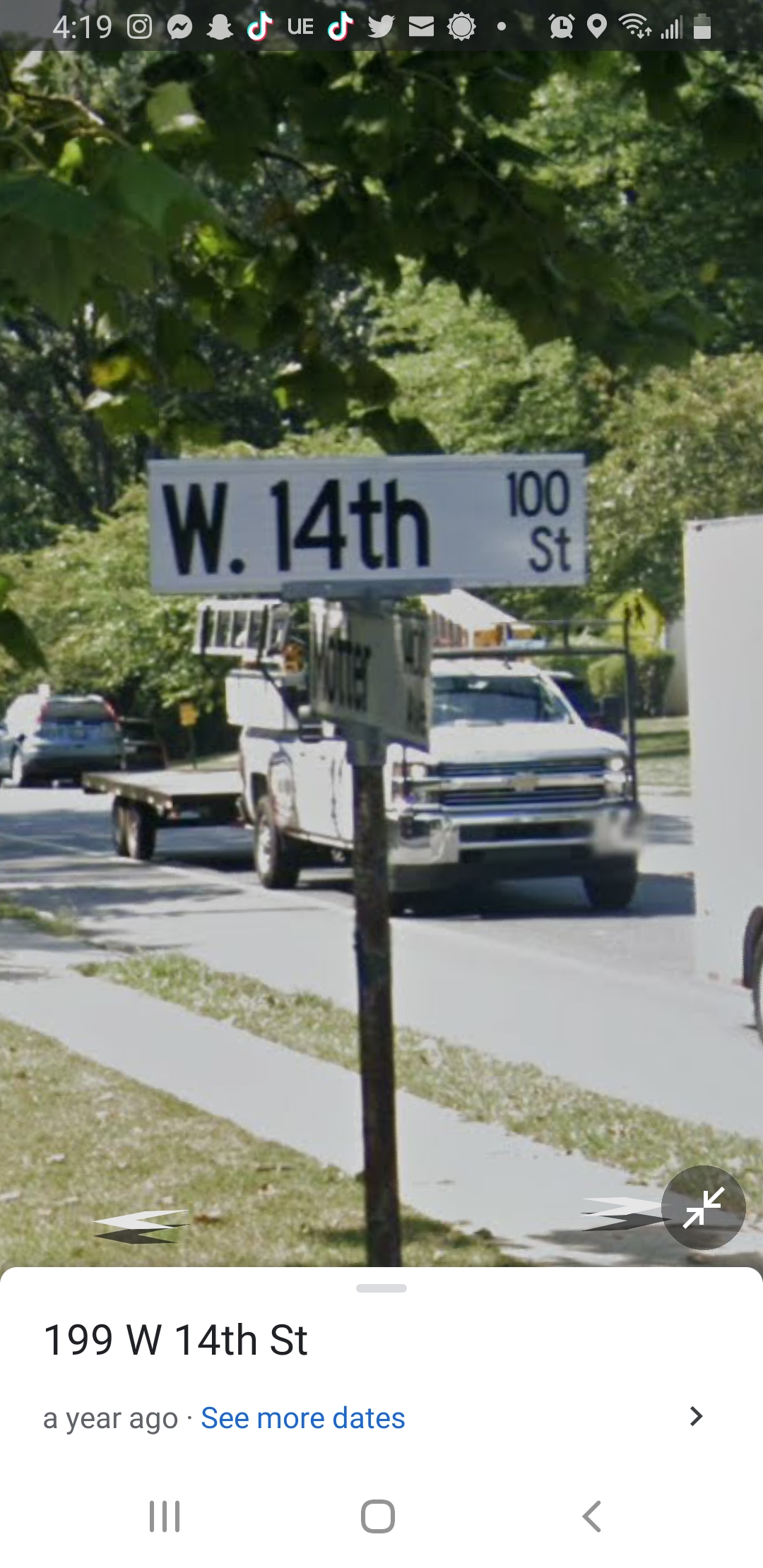This photograph captures a white street sign with black lettering that reads "W 14th 100 ST." Positioned against an urban backdrop, the street sign stands prominently in the foreground. Directly behind the sign, a vehicle with a trailer can be seen, equipped with a ladder secured to its top. 

The uppermost part of the image includes an array of phone screen icons, suggesting the photograph was taken on a mobile device. Along the bottom edge of the photo, the screen display is partially visible and reads "199 West 14th Street," followed by the text "a year ago" and "see more dates." This indicates that the photo was possibly taken and saved on a mobile device about a year prior. The detailed context captured in this image provides a vivid glimpse into a typical urban setting with everyday street infrastructure and a hint of digital interface elements.